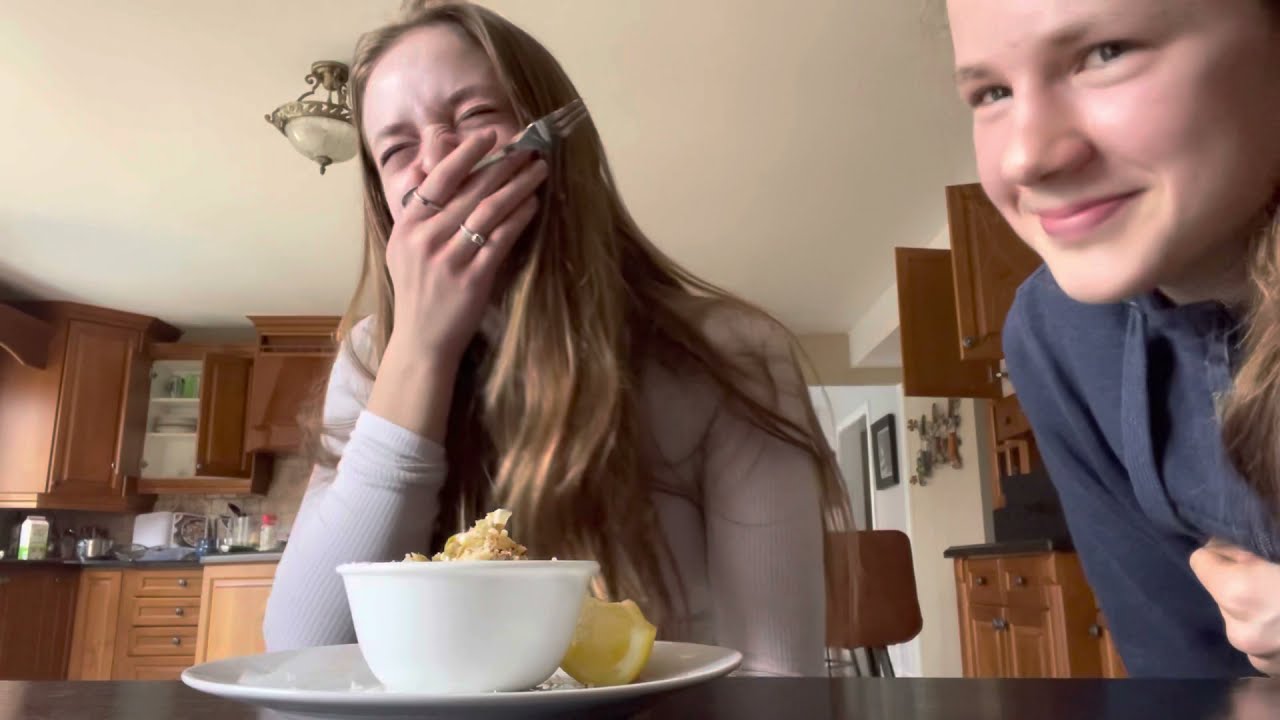This horizontally aligned rectangular picture captures a candid moment of two white women in a cozy kitchen setting. The central focus is on the woman on the left, who has long light brown hair and is wearing a long white shirt. She is laughing heartily with her eyes closed, covering her mouth with one hand while holding a fork in the other. In front of her on the brown kitchen table sits a round glass plate with a bowl that contains some indistinguishable brown object and a lemon slice to the side.

To her right, the second woman, who appears younger and is wearing a navy blue top, is smiling warmly at the camera. Her joyful expression is accentuated by her wide smile with no teeth visible. Only part of her face and upper torso are captured in the frame. The background reveals wooden kitchen cabinets, a sink, and appliances, further adding to the cozy atmosphere. A light fixture hangs prominently from the white ceiling, illuminating the cheerful scene.